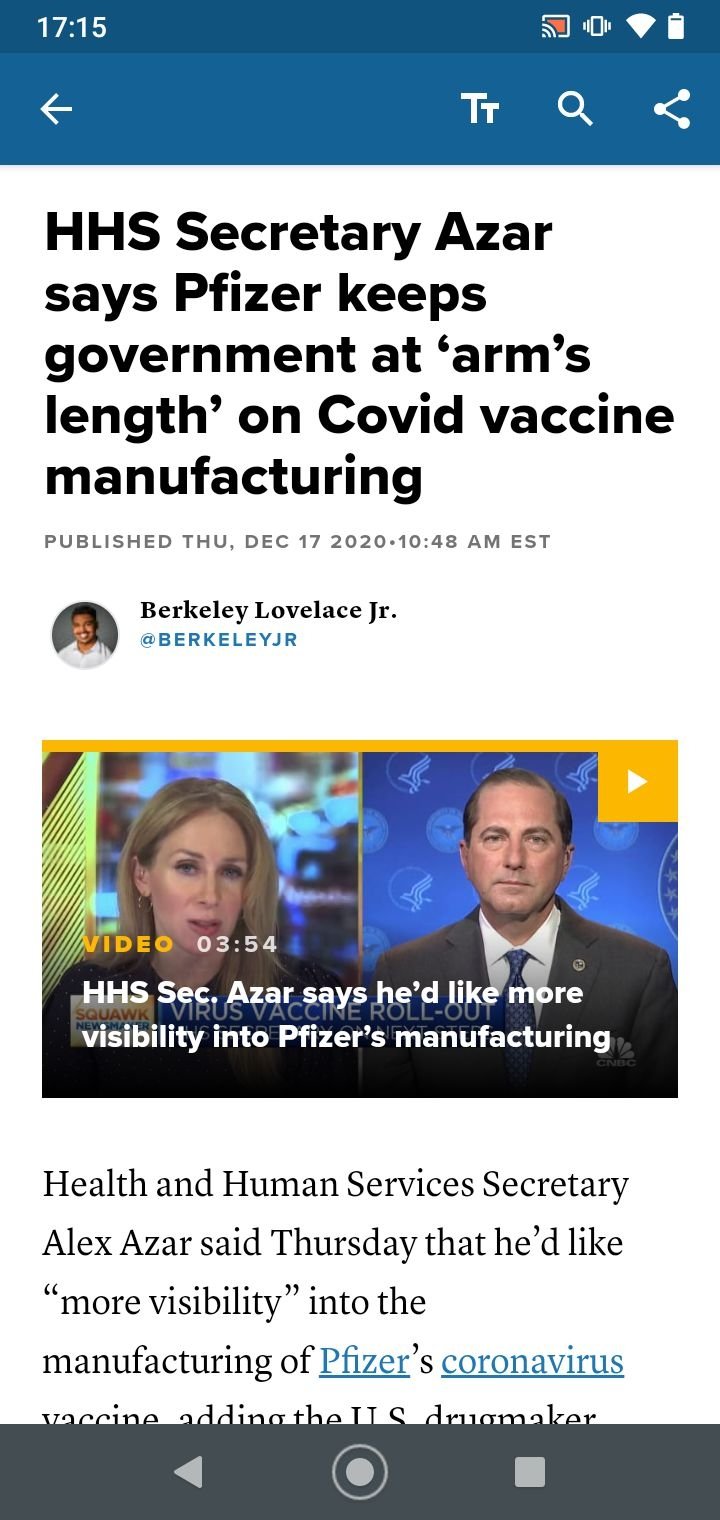This image features a headline at the top, written in black on a white background. The headline reads: "HHS Secretary Azar says Pfizer keeps government at arm's length on COVID vaccine manufacturing," and is accompanied by the publication date "December 17, 2020 at 10:48 a.m. EST." The publisher's name, "Bekele Lovelace Jr.," is written in blue.

Below the headline, there is a video thumbnail. The video information specifies a duration of "3 minutes 54 seconds" and is titled "HHS Sec Azar says he'd like more visibility into Pfizer's manufacturing." The background of the thumbnail features an image of a woman on the left and a man on the right. In the bottom right corner of the video thumbnail, the CNBC logo is visible, while a yellow play button is located in the top right corner.

The accompanying text under the video states: "Health and Human Services Secretary Alex Azar said today that he'd like more visibility into the manufacturing of Pfizer's coronavirus vaccine." Notably, the words "Pfizer" and "coronavirus" are highlighted in blue.